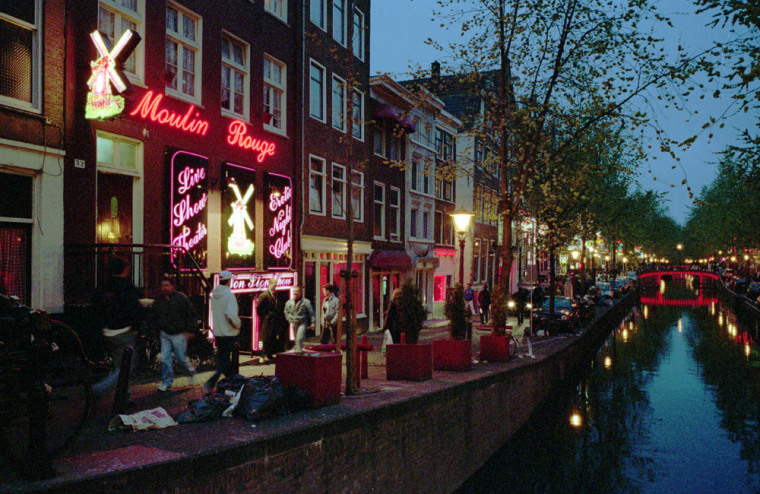This richly detailed photograph, taken outdoors during dusk or nighttime, showcases a picturesque scene reminiscent of Amsterdam. Dominating the right side, a narrow canal stretches away from the viewer, lined with lights on both edges. A stone ledge on the left runs from the bottom left corner, extending up and away, paralleled by a sidewalk. This walkway is bustling with people and flanked by trees, light stands, and a variety of shops.

A standout feature is a prominent building on the left, adorned with a neon sign reading "Moulin Rouge" in red letters. Above its windows, which display purplish neon signs and an image of a rabbit, a picturesque windmill turns gently in the twilight. The canal's path is punctuated by a red-lit bridge in the distance, adding a romantic flair to the scene. Along the street, clusters of pedestrians move in various directions, adding life to the serene, water-bound setting.